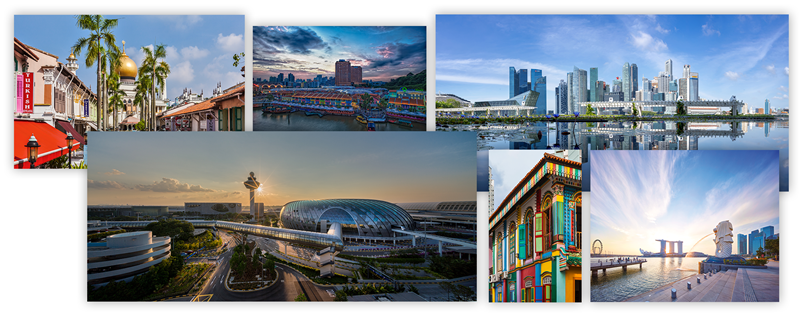This collage features six captivating photographs set against a white or transparent background, showcasing diverse cityscapes. At the top left, there’s an image of rows of buildings interspersed with palm trees and a prominent mosque with a golden dome. Next to it, a smaller snapshot captures a serene waterway with buildings and a vast expanse of sky. The far-right image in the top row displays a bustling city skyline with towering buildings set against a blue sky, fronted by a calm body of water. Overlapping slightly at the bottom, the leftmost photograph highlights striking dome-like and circular buildings under a grayish-blue sky, hinting at modern architecture and possibly a metro link. To its right, there's a vibrant multicolored building. Finally, on the bottom right, a peaceful image depicts a scenic waterfront with a boardwalk, extending serenity and open sky.